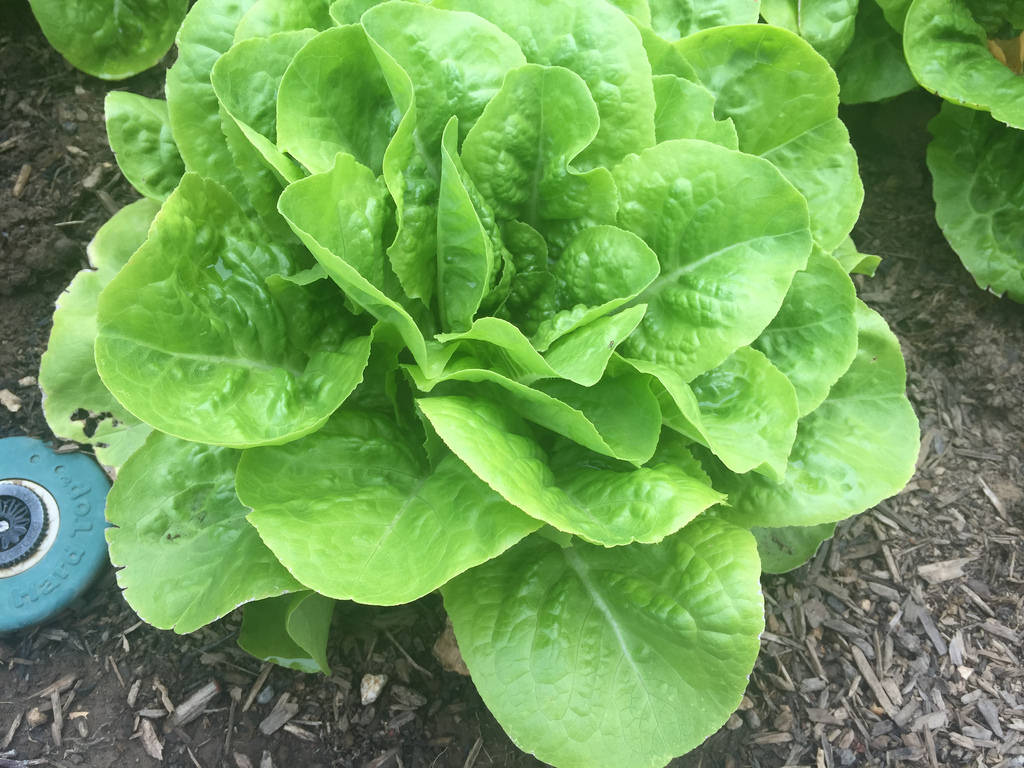In this daytime photograph taken outdoors in what appears to be a garden, the focal point is a vibrant, leafy green plant with large, curvy leaves resembling romaine lettuce. The greens are light and vibrant, with some edges taking on a yellowish hue. The plant is rooted in a mix of grayish, ash-like soil interspersed with small sticks and wood pieces. Prominently visible on the left side of the image is a blue, round device that likely serves as a component of a sprinkler system; it has a plastic encasing with various lines and the partially visible inscription "hand top" on it. Additionally, towards the bottom right of the image, another similar sprinkler component can be spotted. Surrounding the main plant are patches of similar leafy greens, with more plants visible in the background on both the right and left sides. The overall scene captures a detailed and vibrant garden setting, emphasizing the contrast between the lush green leaves and the peculiar soil mixture.